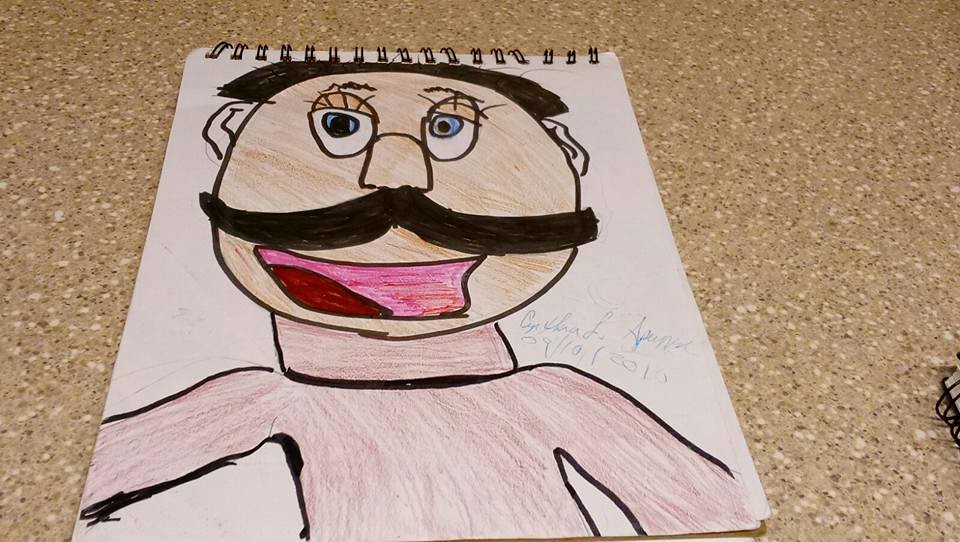In this detailed illustration, a spiral notebook with black rings is prominently displayed on a speckled light brown and beige marble-like table or countertop. The notebook is open to a page featuring a meticulously rendered cartoon character. The character has defined features, such as black hair and small ears outlined in black. The round face is colored light brown, giving it a realistic skin tone, with large, expressive oval eyes shaded blue and accented with black pupils—the right pupil notably larger than the left. The eyelids are delicately drawn and match the light brown hue of the face. 

A prominent feature of the character is a thick, upward-curving black mustache, adding a whimsical touch. The mouth, outlined in black, is filled with shades of pink and red, giving it depth and vibrancy. Below the face, the character has a square-shaped neck colored light brown, followed by partly visible arms and body.

The artist, who signed the drawing with "Cynthia L" followed by some illegible numbers, has captured a balance of cartoonish charm and attention to detail. Nearby on the right side of the image, the top edge of another spiral notebook is just visible, hinting at more creative works lying in wait.